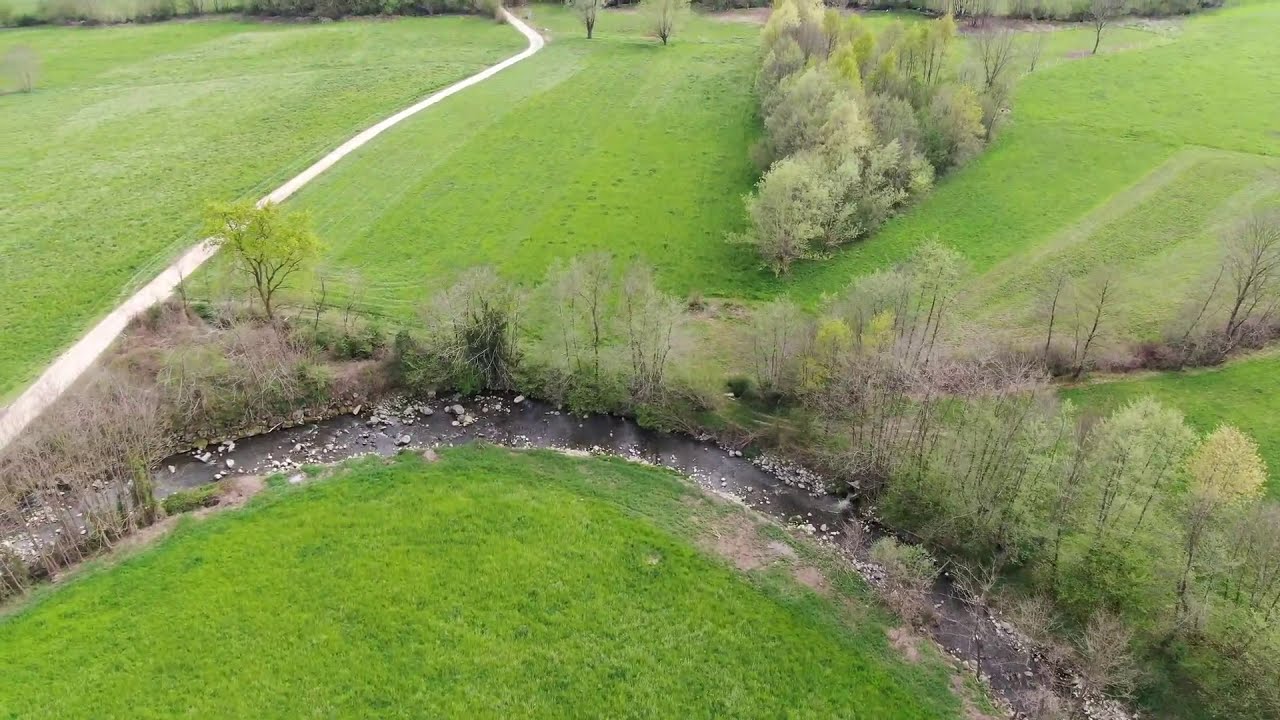This aerial photograph captures a serene countryside scene featuring a prominently curving creek or stream. The waterway meanders from the lower left, arcs up towards the center, then descends toward the lower right, dotted with white and gray rocks that vary in size. On either side of the stream, lush green grasses stretch out, appearing freshly cut and uniformly short. The grassy terrain is interspersed with spindly trees, some resembling aspens, and sparse bushes, which give a sense of early spring as many trees appear lightly leafed or barren.

A notable feature of the landscape is a narrow white path made of gravel or limestone. It begins from the middle left and winds gently uphill towards the center top of the image before veering slightly left again. This pathway traverses through the grassy expanse, suggesting it's a well-trodden walk for visitors, perhaps within a park. The lower portion of the photograph highlights a grassy area shaped somewhat like the top of a circle, around which the creek curves.

In the backdrop, beyond the initial bend of the creek, lies more spreading grassland with additional trees and another bend of the creek meandering into the distance, enhancing the tranquil and picturesque nature of this aerial countryside view.